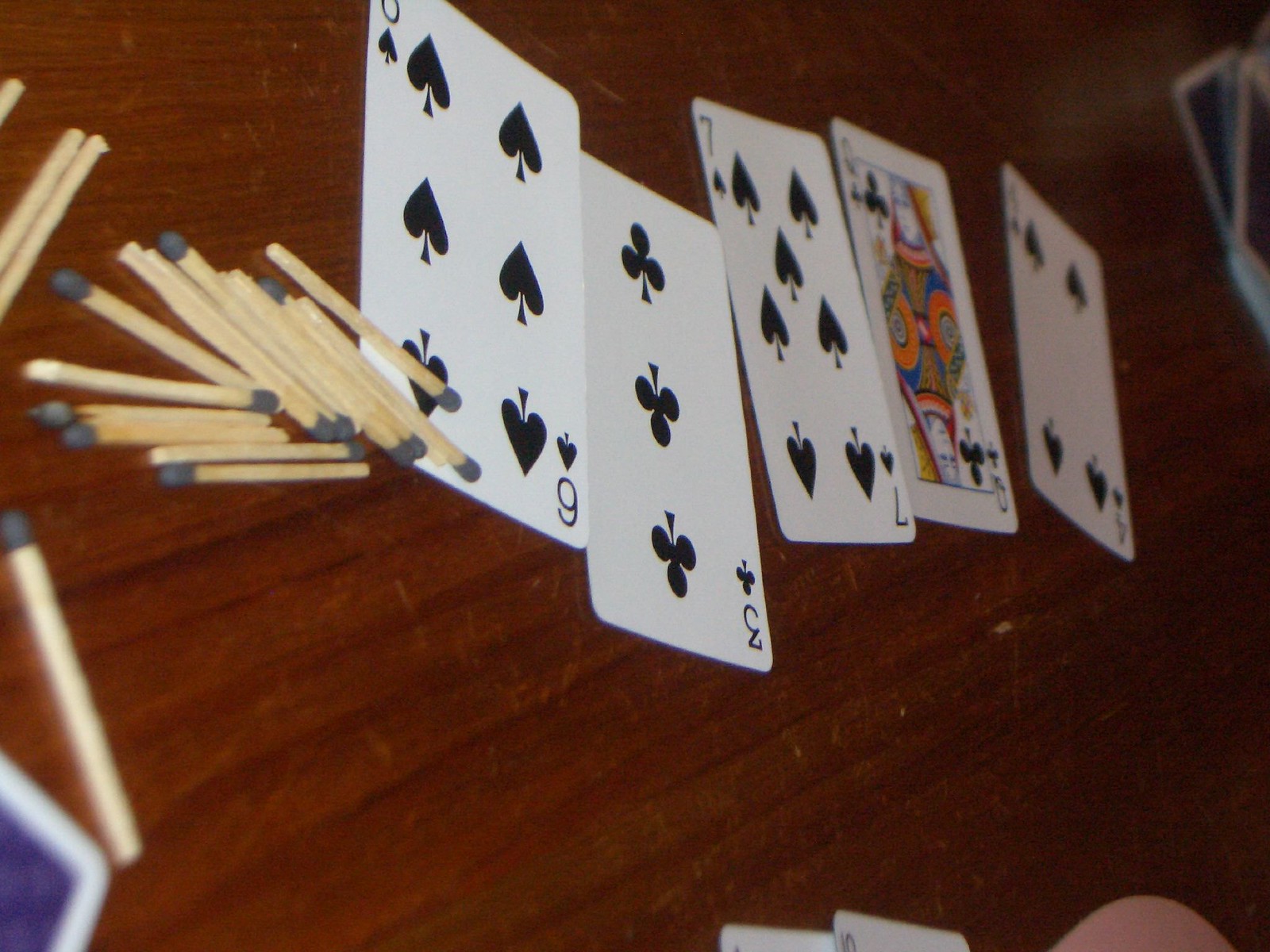This close-up photograph captures an intriguing arrangement of playing cards and matches on a dark, reddish-brown wooden tabletop. The focal point is a neat row of five playing cards: from left to right, they are the six of spades, three of clubs, seven of spades, queen of clubs, and four of spades. The cards are organized in a straight line, clearly showcasing their values and suits.

To the left side of the image, a scattered pile of wooden matches lies haphazardly on the table. These matches appear to be used, as their heads are a greyish-black color, indicative of having been burnt, although the sticks themselves remain relatively clean. Some of the matches touch the bottom left corner of the six of spades, creating an interesting visual connection between the cards and the matches.

In the bottom left corner, a small fragment of another card is visible, though it's flipped to show its back side. At the bottom edge towards the right, a portion of a person’s flesh – possibly a hand, knee, or elbow – subtly enters the frame, adding a human element to the scene. To its left, the edges of two more cards peek into the shot, though their identities remain a mystery. Lastly, in the top right corner, a small stack of upside-down cards can be seen, with only their backs showing. The photograph is rich in texture and detail, inviting viewers to linger and explore the nuanced interactions between the various elements.